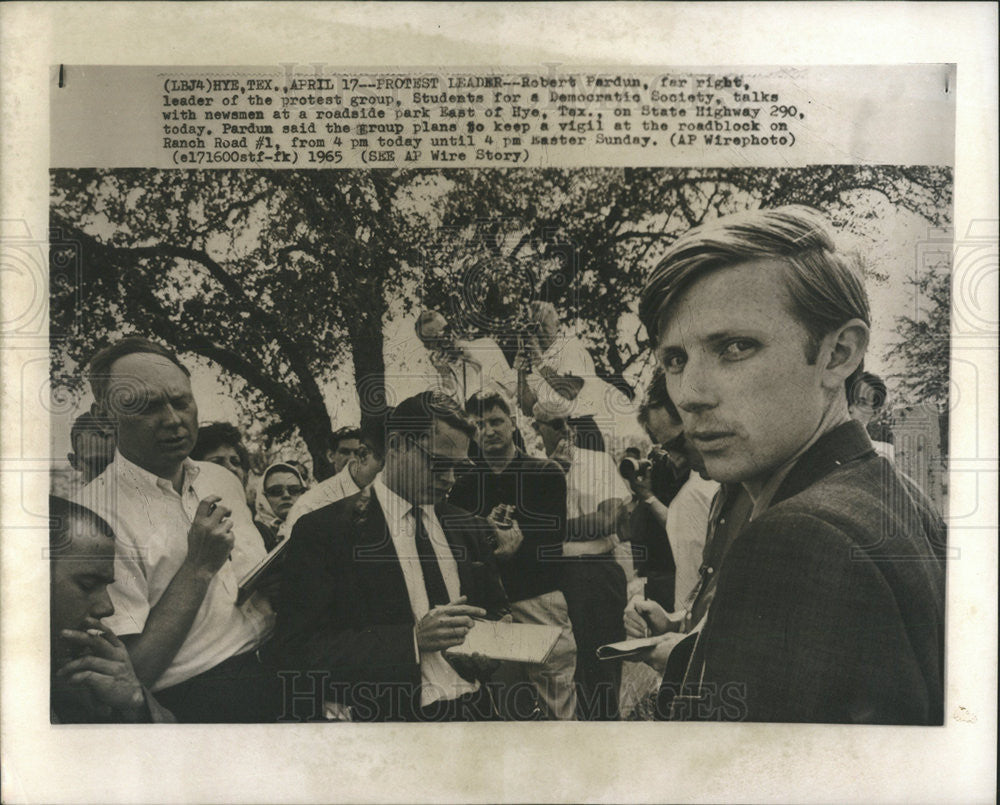This image, a cutout from a 1965 newspaper, captures a gathering of predominantly men in suits and ties, with a few women in the background, at a roadside park east of HYETEX on State Highway 290. The central figure, Robert Pardum, far-right leader of the protest group Students for a Democratic Society, stands prominently on the right side of the image, directly facing the camera with a serious expression. Around him, several men—some holding notebooks or cameras, others appearing engaged in conversation or smoking—focus their attention either on Pardum or on their notes. Among the crowd, people are seen writing or referring to their books, suggesting the presence of journalists or newsmen. A tree is visible in the background, adding a touch of nature to the scene. At the top of the image, the caption reads "LBJ4, HYETEX, April 17th," followed by a description of the ongoing event: Pardum discussing plans to maintain a vigil at the roadblock on Ranch Road No. 1 from 4 p.m. today until 4 p.m. Easter Sunday. The notation "(PYR photo)" and the year 1965 further authenticate the historical context of the photograph.